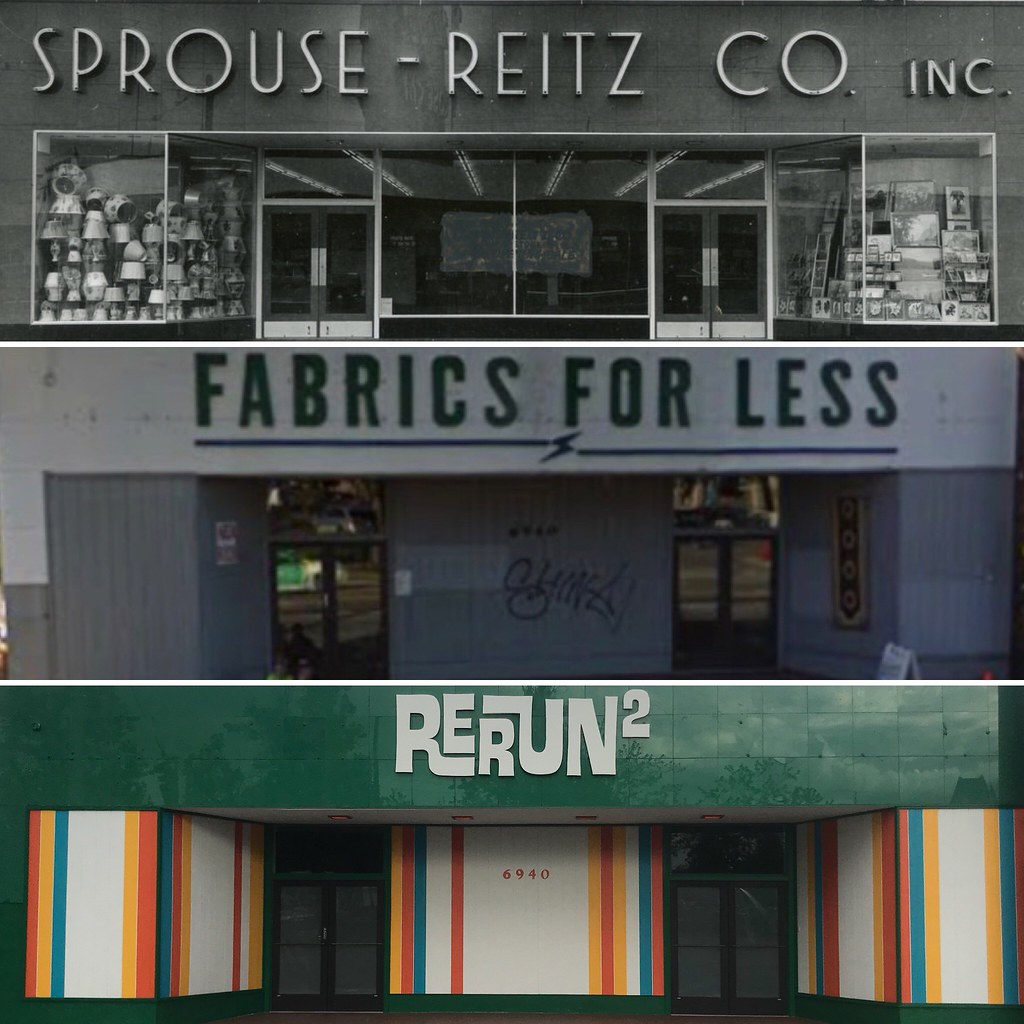The image showcases three distinct storefronts, each with unique characteristics. The top storefront is depicted in a black-and-white image and is labeled "Sprouse-Reeds Co. Inc." The frontage features two prominent doors flanked by ample glass windows, displaying various items. On the left side of this display area, there are lampshades, while the right side showcases diverse picture frames.

The middle storefront is identified by the green sign "Fabrics for Less." Below the sign are glass doorways, with gray sections in between. One of these gray areas is adorned with graffiti. The sign includes a blue lightning bolt line underneath it, set against a white wall.

The bottom storefront has a vibrant green background with the name "Rerun 2" written in a funky, stylized font. Below this sign are two glass entranceways. The adjacent white walls feature colorful strips of orange, yellow, and blue. Centrally located above this storefront is the number "6940."